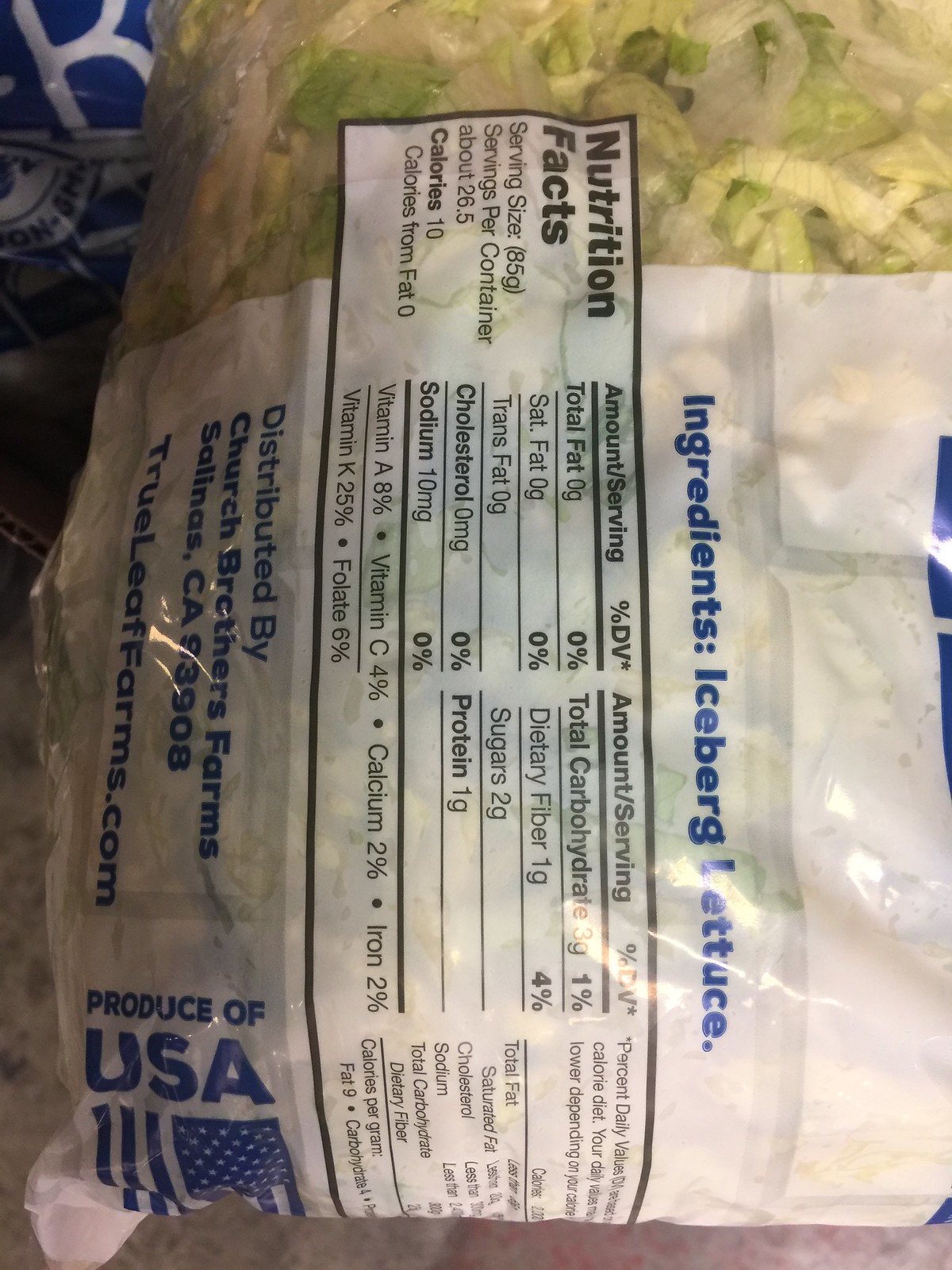This photograph captures the back of a food package, specifically designed for iceberg lettuce. The package is made from clear and partially transparent plastic. Dominating the back is a white rectangular section featuring the "Nutrition Facts" in bold, black text. The image is rotated at an unconventional angle, causing the text to appear sideways. Below the nutrition information is another white section with blue text, listing the sole ingredient: "Iceberg Lettuce." The clear packaging reveals the contents, showing pre-shredded iceberg lettuce inside.